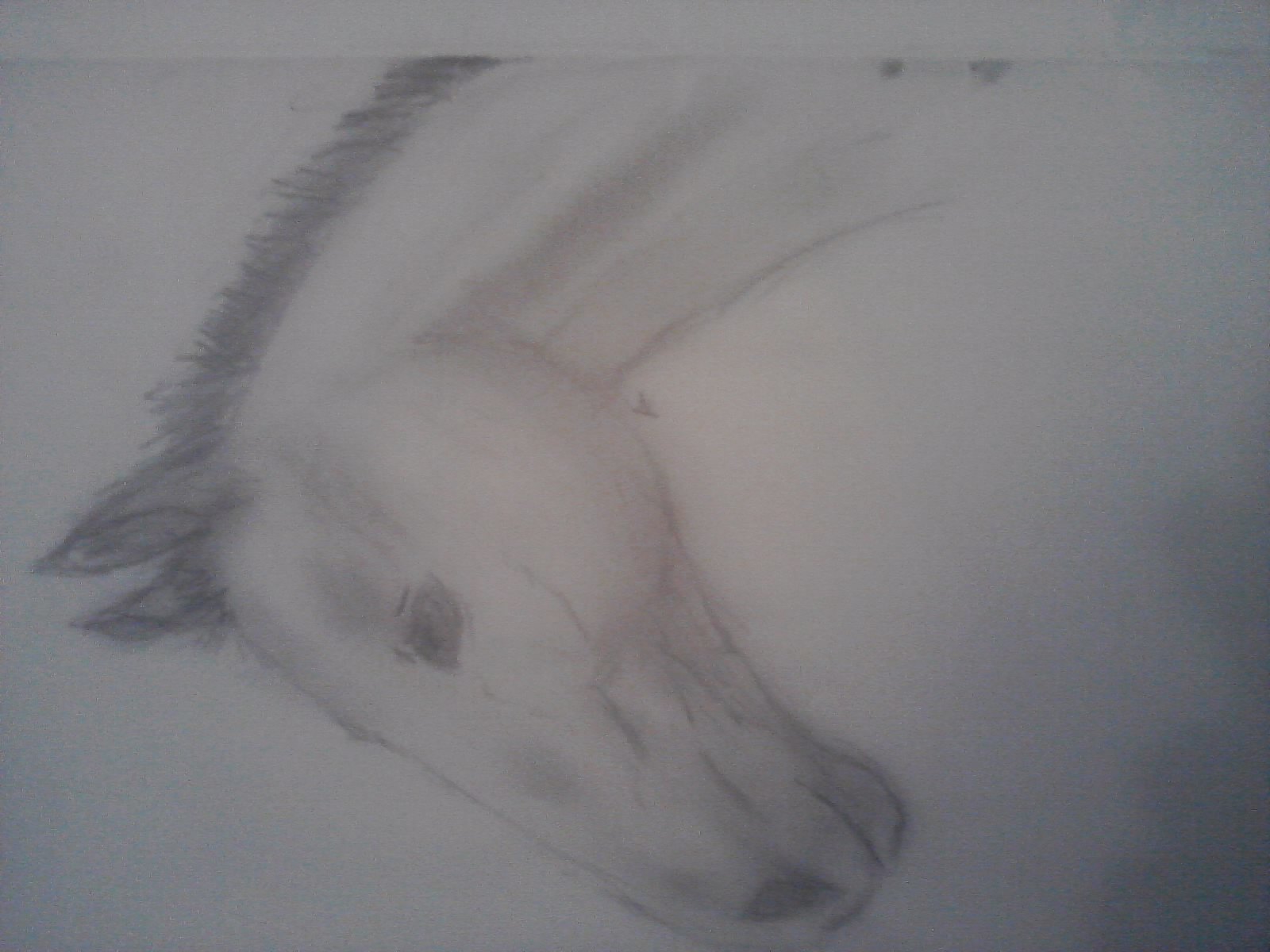A detailed pencil line drawing of a horse's head and upper neck displayed on a white sketchpad has been rotated 90 degrees counterclockwise, presenting the horse's profile to the viewer with its head pointing downward and neck extending upward. The ears are pointing to the left, while the mane appears diagonally across the top. Fine details such as the eyes, ears, nose, and mane are prominently shaded, capturing the essence of the horse with subtle shading on the veins, mouth area, nostrils, and underneath the neck. This sketch is recognized for its clarity and immediately identifiable depiction of a horse, set against some shadow casting in the bottom right corner, contributing to its depth and realism. The simplicity and effectiveness of the line work suggest meticulous craftsmanship, even though the overall style leans towards minimalistic rather than overly detailed.